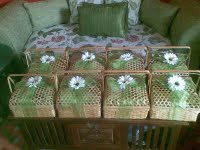This detailed, color photograph captures a cozy indoor scene. Centered in the image are eight light brown wicker baskets, each fitted with a wicker lid and adorned with a white flower that has a striking black center. The flowers are tied to the baskets with clear or opaque green ribbons. These baskets rest on a dark wooden coffee table characterized by its multiple dark brown supports that connect to a square base featuring intricate engravings.

In the background, a plush olive green sofa takes up the backdrop. The sofa is complemented by darker green silk pillows and a rectangular green pillow. Draped over the sofa is a blanket that functions as a throw, its white fabric embroidered with pink and red flowers and green leaves. The seated portion of the sofa showcases a white fabric with a matching green and pink floral print, adding a touch of elegance to the cozy setting. The photograph, taken in landscape mode, skillfully captures the intricate details and harmonious color palette of this inviting living space.